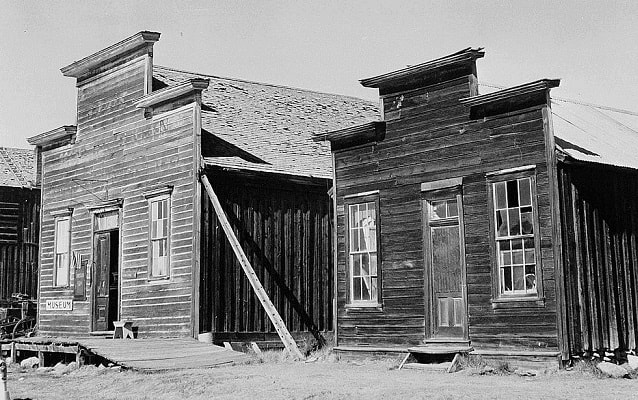This black-and-white vintage photograph captures two quintessential Old West USA style wooden buildings. Both structures feature square front facades composed of horizontal wood slats, with vertically aligned wood on the sides. Each building has a typical triangular-shaped, tiled roof and boasts two sash windows flanking a central wooden door. The building on the left, slightly larger, has a wooden plank ramp leading to a small porch in front of the door, and prominently displays a sign that reads "Museum." In contrast, the smaller building on the right has a darker exterior and wooden steps that elevate the entrance, presumably to guard against mud during the rainy season. The scene is set on a dirt road, with scattered rocks at the base of each building, enhancing the authenticity and historical ambiance of the Old West town.